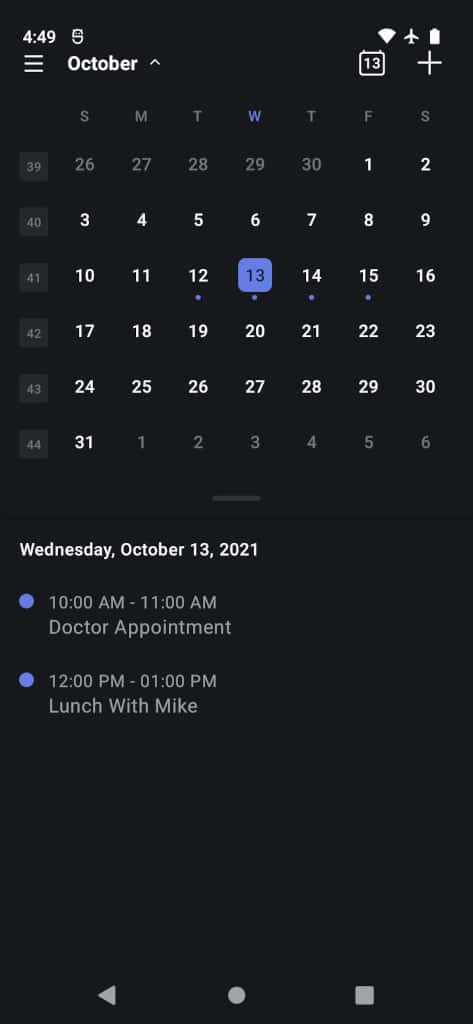A smartphone screenshot captured at 4:49 PM. The status bar displays strong Wi-Fi signal, airplane mode activated, and a full battery. The screen shows a calendar for October, accessible via a drop-down menu. The calendar starts on a Friday, October 1st, and ends on Sunday, October 31st. The last five days of September and the first six days of November are also visible. The date October 13th is highlighted with a blue box. Below the calendar, the text "Wednesday, October 13th, 2021" appears in white. Further down, two event entries are listed: "10 a.m. - 11 a.m. Doctor's Appointment" and "12 p.m. - 1 p.m. Lunch with Mike," each beside a blue circle. At the very bottom are three buttons for additional options.